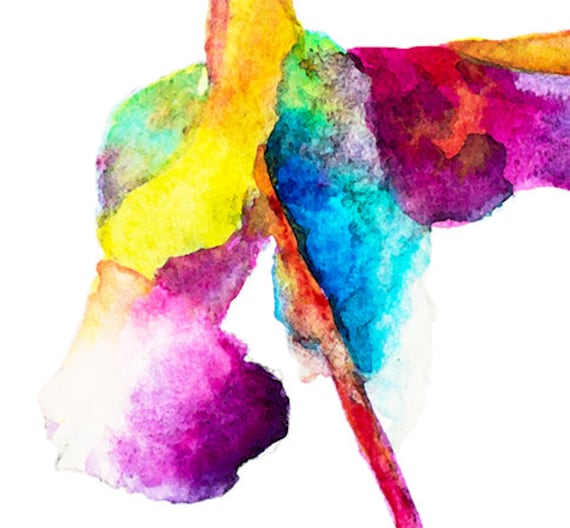The image showcases a vibrant, abstract composition resembling a watercolor painting with no discernible objects. In the bottom left corner, there is a vivid pink and purple blob, radiating a sense of energy. Above it, a yellow blob vaguely resembles the lower part of a horse's leg. Directly above this, a multi-hued mixture of green, blue, and pink paints another indistinct form. Diagonally extending from the "horse leg" shape is a downward red streak, leading to the bottom of the image. Atop this red shape, there's a blue blob, lending a cool contrast. The upper right section features another pink and purple blob, accompanied by a small yellow spot above it. The watercolor-like splotches sit prominently against a stark white background, enhancing their bright, chaotic appearance.